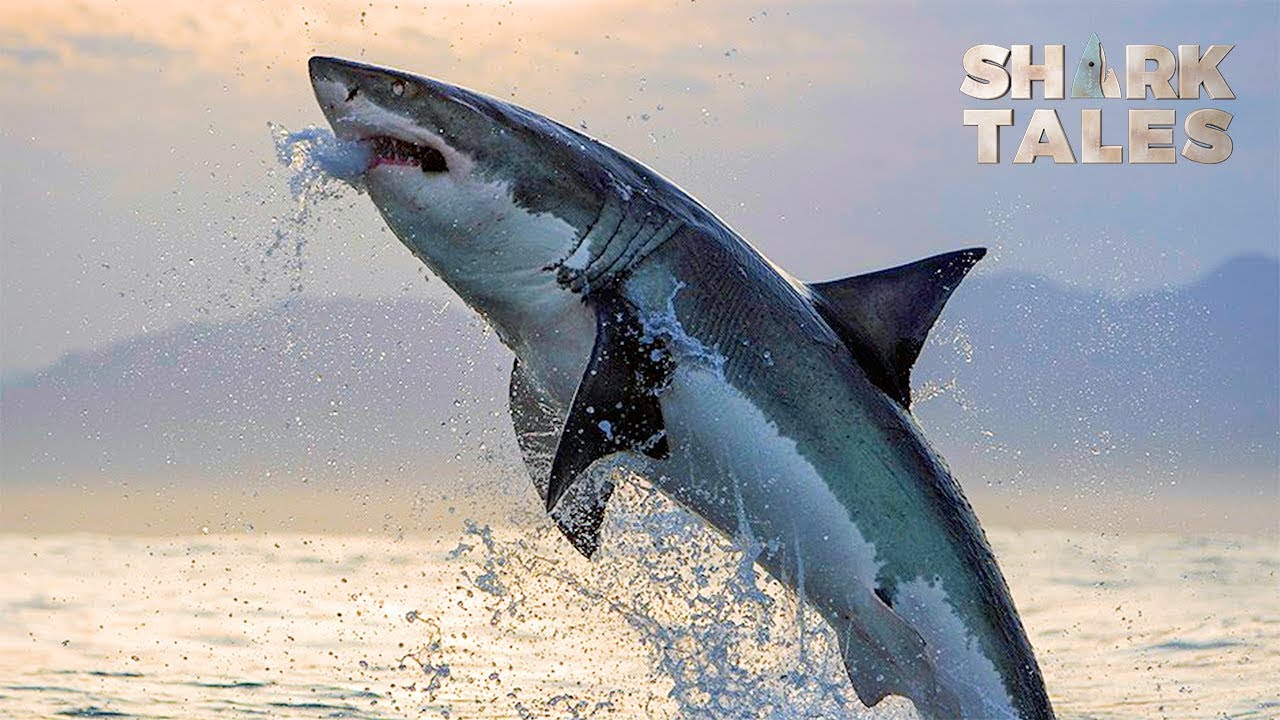The image vividly captures a great white shark leaping out of the water, oriented from the lower right towards the upper left. The shark's body is dark gray or black on the back and white on the underbelly, with water spilling from its seemingly closed mouth. It appears to have something in its mouth, possibly a fish, though this is obscured by the water. The sunlight reflecting off the water below creates a shiny, whitish-yellow hue. The shark's realistic features, including its jagged teeth and distinct fins, add to the dynamic scene. In the background, a mountain range or large hill is silhouetted, enhancing the natural setting. Over this dramatic scene, the top right corner of the image features the text "SHARK TALES" in light copper-colored letters, each on its own line. Notably, the 'A' in "SHARK" is stylized as a shark head facing upwards. The sky above these elements is a blend of blue with a hint of pinkish clouds, adding a touch of color to the striking composition.